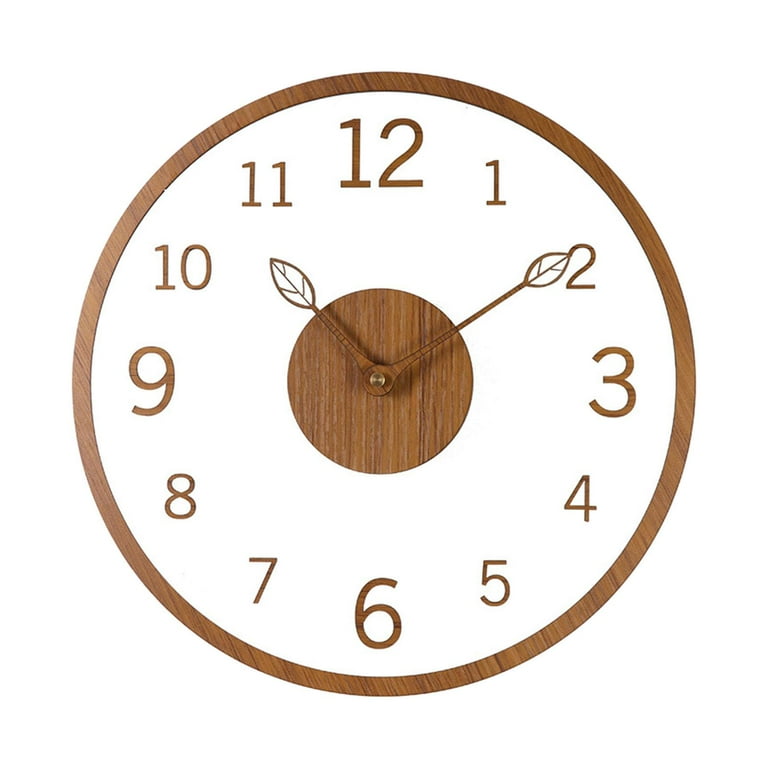This image depicts a modern, artsy wall clock with a wood-themed design. The clock features a light brown wooden border that encircles a white plastic background. At the very center of the clock is another wooden circular element. The clock hands, designed to resemble tree branches, have transparent leaf tips with detailed inner veins. The hour markers are etched into the white background, with the 12, 3, 6, and 9 significantly larger and more prominent than the others. The remaining numbers are smaller but equally wood-themed. The minute hand is currently at the 2, while the hour hand rests between 10 and 11, indicating a time of approximately 10:10.